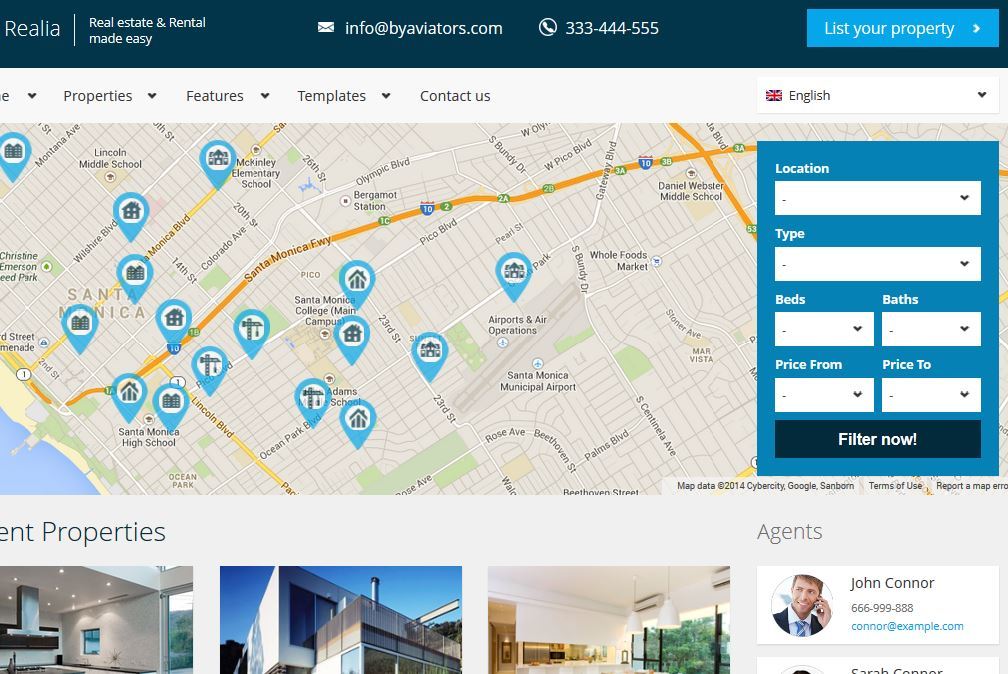In this image, we see a detailed view of a real estate and rental website. At the top left, the company name is displayed alongside the slogan "Real Estate and Rental Made Easy." Below this, contact information is provided, including the email address info@buyaviators.com and the phone number 333-444-555. 

On the top right of the webpage, there is a menu with options such as "List of Property." Below these elements, a map highlights various locations, including notable areas such as Colorado Avenue, Lincoln Blvd, Ocean Park Blvd, Santa Monica High School, Wishart Blvd, McKinley Elementary School, Lincoln Middle School, and Olympic Blvd.

To the right of the map, information about emergency locations is provided along with filters for type of property, number of beds and baths, and a form for price range. This ensures that users can easily find and sort properties according to their preferences.